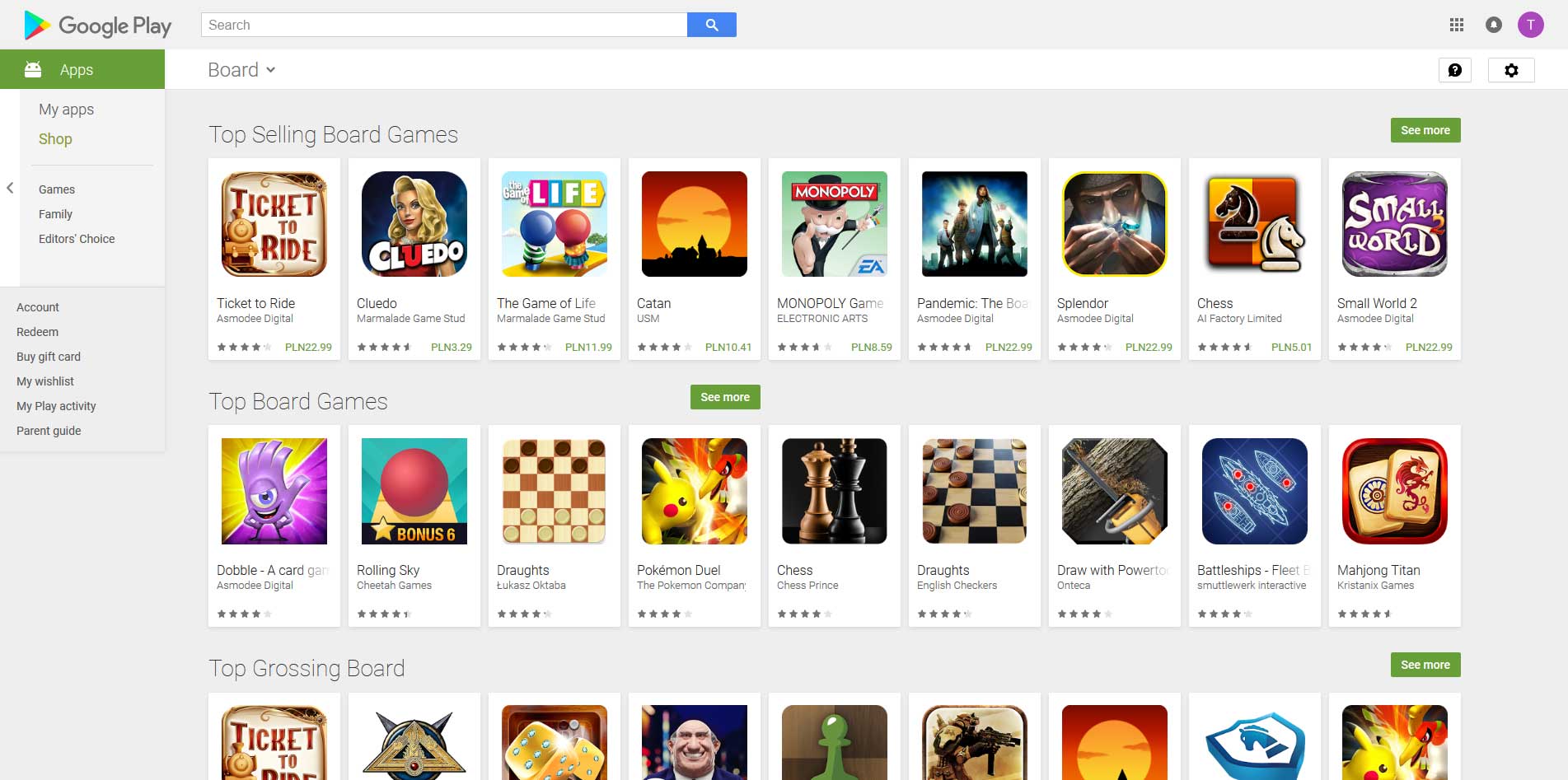A detailed screenshot from the Google Play Store app is depicted, featuring a grey background with the Google Play logo prominently displayed at the top left corner. Centrally positioned is a search bar adorned with a blue magnifying glass icon. To the left of the search bar, a menu listing several sections such as "Apps," "My Apps," "Shop," "Games," "Family," and "Editor's Choice" is visible. Another submenu beneath this provides options for "Account," "Redeem," "Buygift.com," "My Wishlist," "My Play Activity," and "Parent Guide."

The user has selected the "Board Games" category, and the display shows the top-selling board games available on the Google Play Store. The screen reveals two full rows, each containing nine game icons, alongside their titles and thumbnail images. The games listed include:

1. Ticket to Ride
2. Cluedo
3. The Game of Life
4. Catan
5. Monopoly
6. Pandemic
7. Splendor
8. Chess
9. Small World 2
10. Dobble
11. Rolling Sky
12. Draughts 
13. Pokemon Duel
14. Another Chess game (duplicate mention likely)
15. Another Draughts game (duplicate mention likely)
16. Draw with Powerton
17. Battleships
18. Mahjong Titan

Partially visible are additional game icons, suggesting more options further down. Each game icon features a distinctive advertisement image representing the respective game, giving users a quick visual reference.